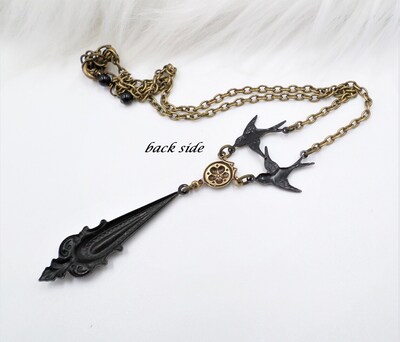The image depicts an intricately designed necklace with a gold chain, positioned on an off-white surface. The chain appears to weave left to right and back across the image, with black accents, possibly small balls, near the top. At the point where the chain converges, there are two swallows or doves holding up a circular section adorned with a petal motif. This motif supports a teardrop-shaped pendant that bears a dark metallic hue, which seems to be leaf-themed. The necklace appears somewhat antique, displaying a blend of black, light gold, and off-white colors. The uppermost section of the image features what looks like short white hair or fibers, which could be from fabric, carpet, or human hair. Additionally, black text on the left side of the chain reads "back side." The photograph captures a meticulously detailed view, highlighting the elegance and age of the jewelry against its neutral backdrop.